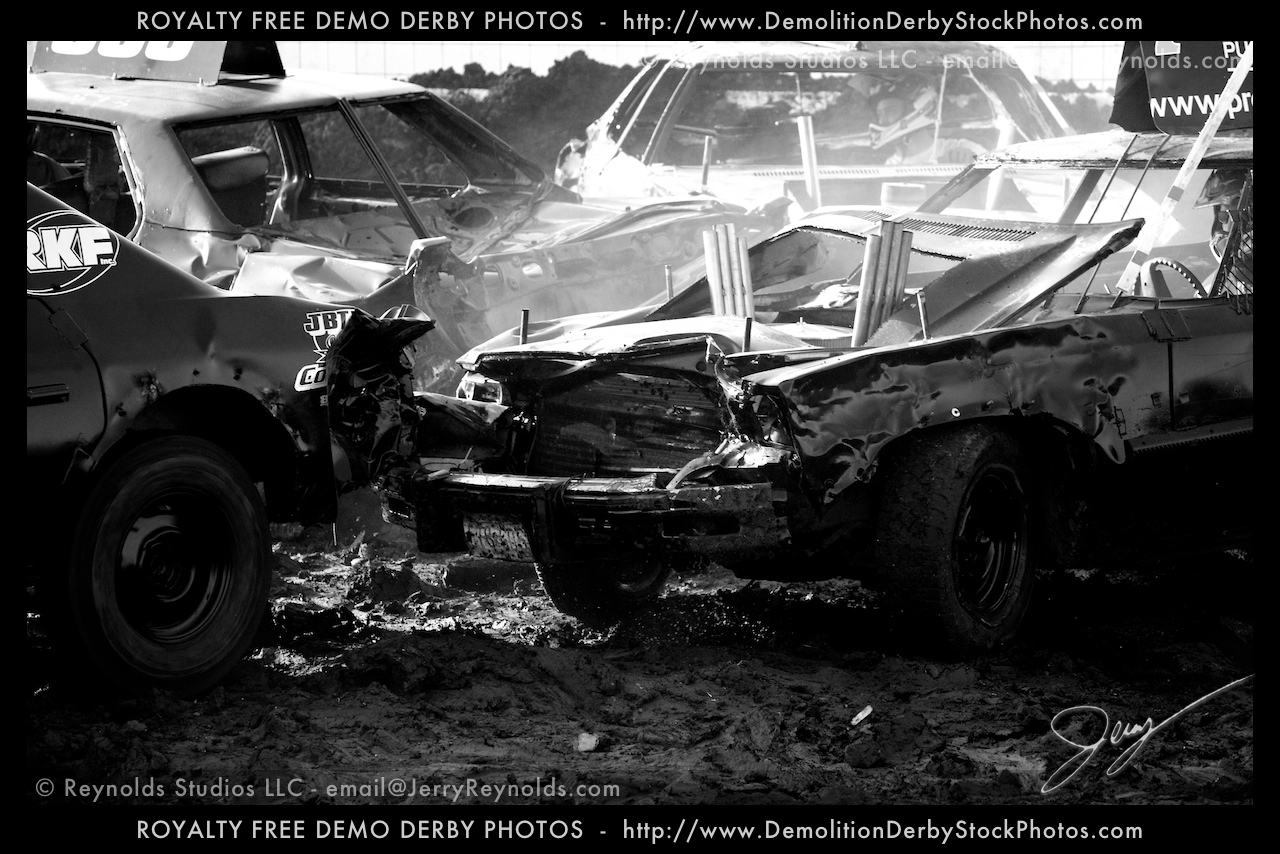This black-and-white photograph showcases the aftermath of a demolition derby, featuring four heavily damaged cars positioned in a muddy lot. At the top of the image, a black border with white text reads "Royalty-Free Demo Derby Photos," along with the website "demolitionderbystockphotos.com." The bottom border of the image also displays this information, alongside the copyright notice "Reynolds Studios LLC" and a contact email "jerryreynolds.com." A cursive signature, likely "Jerry," is visible in the bottom right corner.

The photograph itself highlights a chaotic scene: four cars in various states of disrepair. The car in the forefront has a completely smashed front end, with the hood missing and the windshield bashed in, exposing the steering wheel. Another car, distinguishable by an "RKF" symbol on the back, has a severely crushed rear end, suggesting a violent collision. Additional cars in the background exhibit similar extensive damage, with dented bodies, lost roofs, and shattered windows, all reinforcing the image's dramatic documentation of a demolition derby.